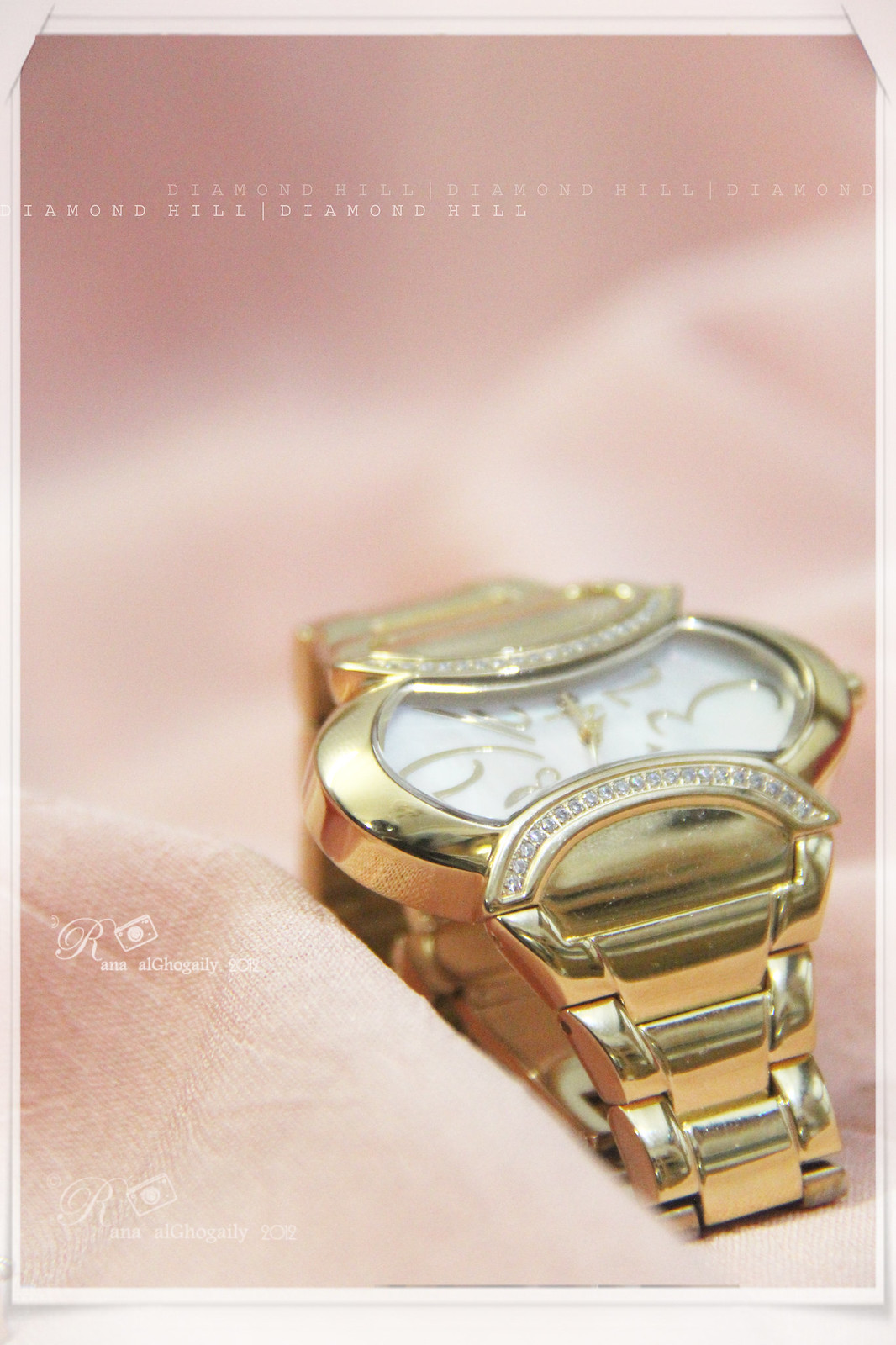The image features a light pink or rose gold fabric background, which appears to be silk. The top of the image includes the text "Diamond Hill" in faint print, with a slightly brighter white ‘Diamond Hill’ printed twice below it. At the center of the image, there's a luxurious gold wristwatch. The band of the watch widens progressively as it approaches the watch face, which is protected by a glass cover. The watch face is white with gleaming gold numbers and hands. Enhancing its opulence, the watch has an arch of diamonds positioned at both the top and bottom of the face. The gold band is designed with an interlocking chain motif. Notably, in the bottom left corner of the image near the watch, there is text that reads "Rana R-A-N-A-L-G-O-G-A-L-E 2012."